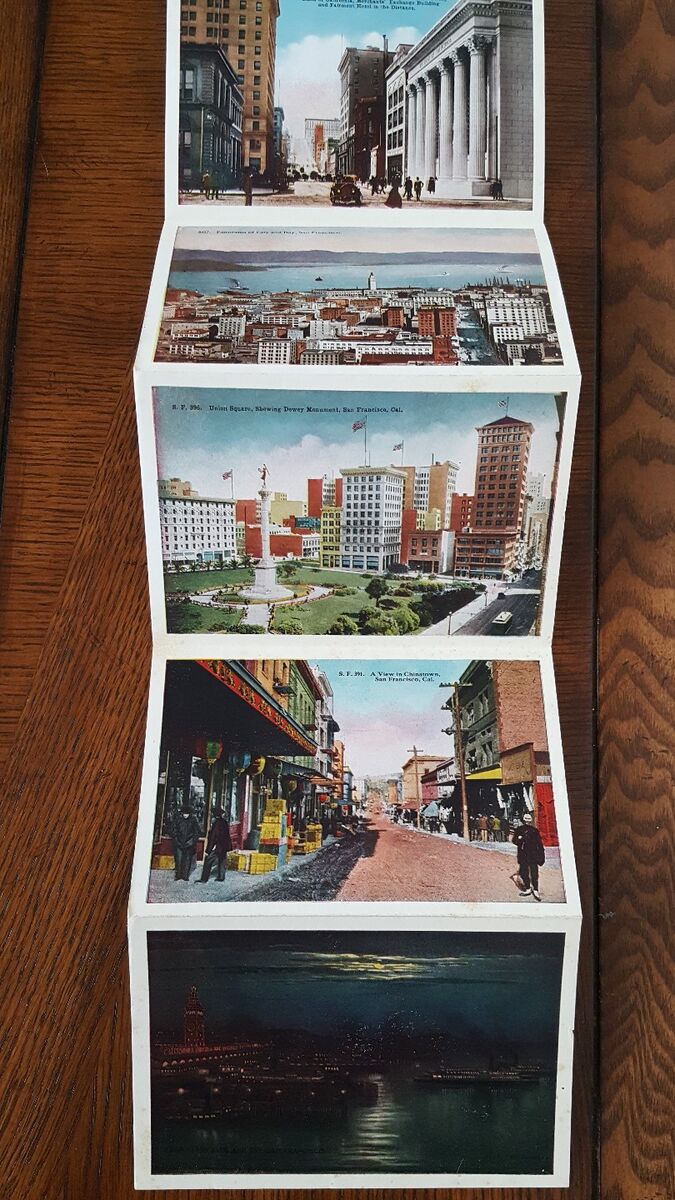The image depicts a vintage folding photo album or postcard strip, dating back to the 1960s or 70s, featuring five small, interconnected photographs that unfold in an accordion shape. Each photograph captures various cityscapes and locations, suggesting popular tourist destinations. The top image showcases a view of a city street, featuring a notable white building with pillars and what looks like a hotel in the background. Below, the second photograph offers a sky view of another city, and the third image highlights a park or fountain amidst urban buildings. The fourth picture provides a glimpse of a bustling marketplace, possibly a Chinatown area, and the last photograph captures a nighttime cityscape with a reflective lake under a setting sun. The entire strip is laid out on a flat surface, likely a coffee table, emphasizing its nostalgic and vintage appeal.